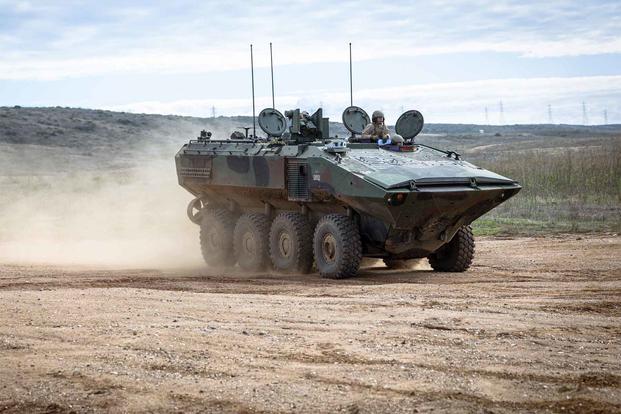This horizontal, rectangular color image showcases a large, dark green amphibious half-track vehicle with a camouflage design, moving from the left to the right across a sandy, desert-like terrain. The vehicle features a distinctive tapered front, resembling an axe head, and is equipped with four thick wheels on each side, designed for traversing various types of soil. The vehicle's slightly upward-tapered front creates a mouth-like appearance. At the top, several turrets are visible; one turret in the upper right hosts a soldier with his head and upper body emerging outward, wearing a light brown helmet and uniform. He appears to be vigilant, looking straight ahead. Behind the half-track, plumes of light brown dust or sand are being kicked up as it advances. The background includes low-lying hills and sparse shrubs, with a clear blue sky filled with wispy clouds overhead. A dirt road is visible leading towards the upper right center of the image.